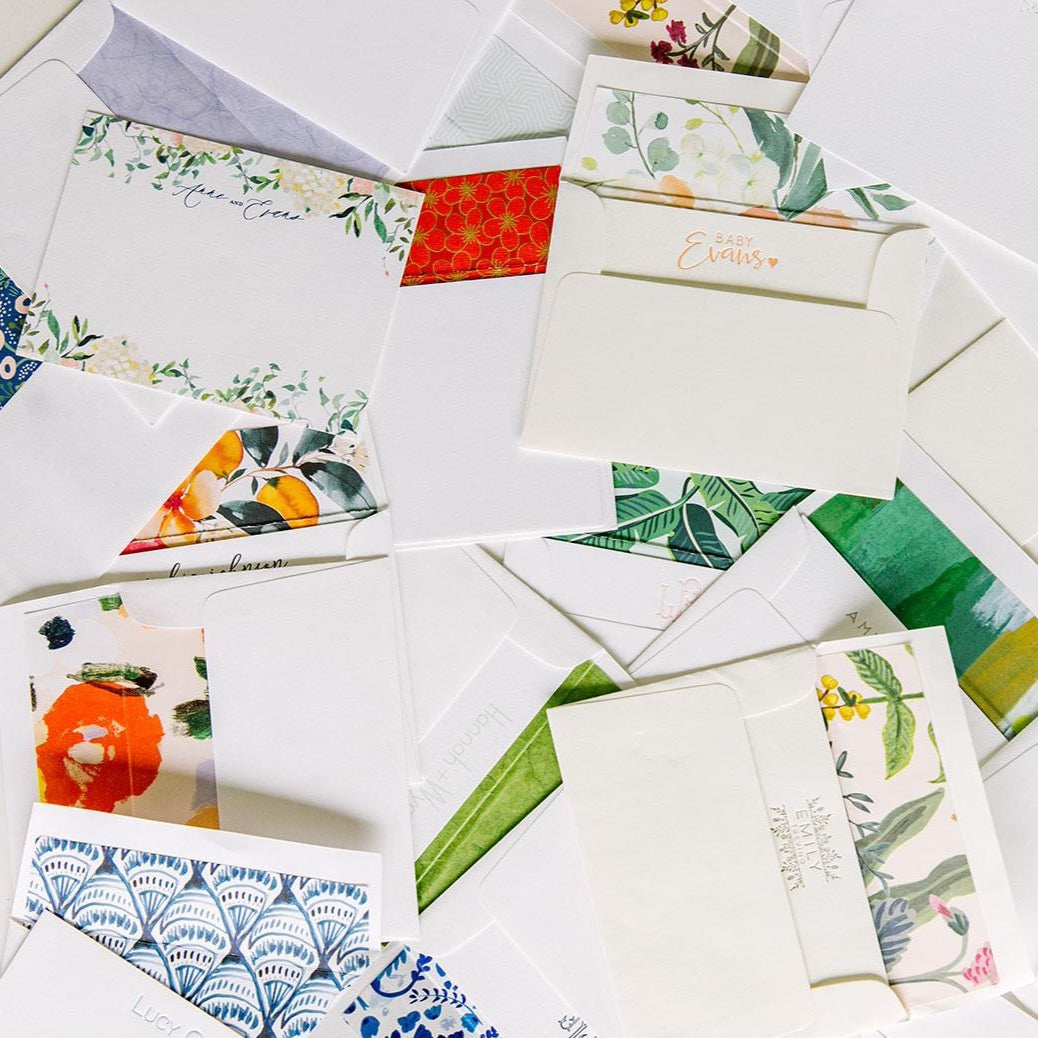The image depicts a messy display of greeting cards and envelopes spread across a white table. The cards are draped in various directions, some stacked and overlapping others. Each greeting card comes with its own envelope, some of which are open while others are closed. The cards themselves feature a variety of designs, predominantly plant-related, and showcase simple images with a color palette of mostly light green and light blue. There are also splashes of other colors including blue on the lower left, red in the upper center, and orange and green on the right and lower center. Specific envelopes are visible, one labeled "Baby Evans" and another "Emily." Among the assortment, a bright orange card that might depict a pumpkin with a hat is notable. The cards appear to be blank, providing ample space for personalized messages, suggesting they are meant for various occasions such as birthdays, anniversaries, and parties.